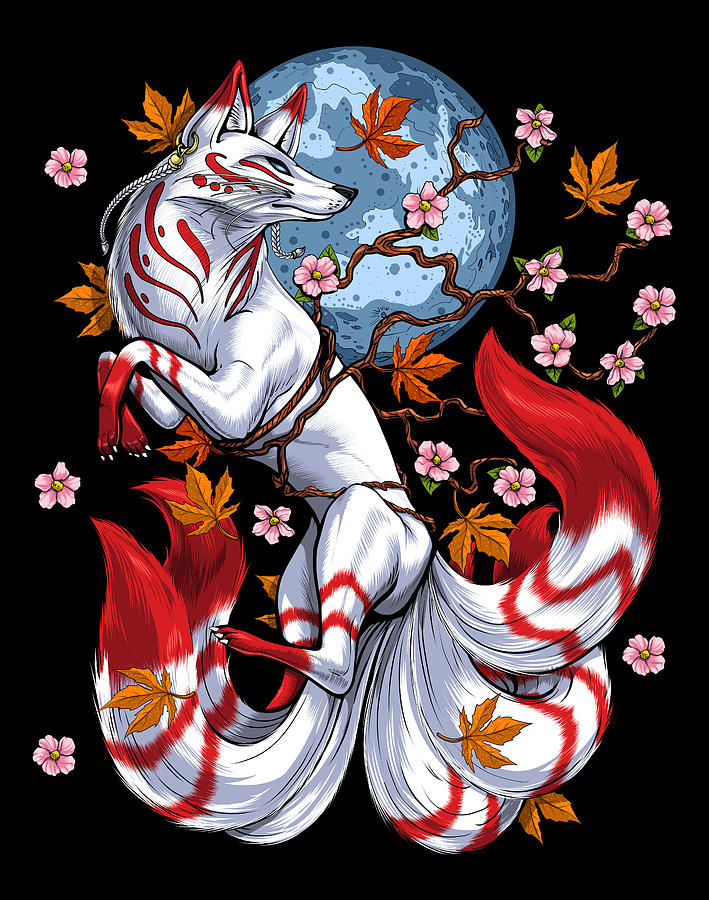This illustration features a striking mythical fox-like creature with detailed anime-style artistry. The central figure is a majestic white fox with an elaborate tail structure, comprising five expansive tails that extend in various directions. Each tail is adorned with red stripes and culminates in vivid red tips. The fox's fur is predominantly white, accentuated by intricate red markings on its face, neck, and paws, resembling red socks. Its face displays blue eyes, a black nose, and ears that are white at the base with red tips.

The creature is depicted looking to the right, though its body is oriented towards the left. It stands against a dark backdrop dominated by a large, blueish-gray moon or globe, enhancing the mystical aura of the scene. Surrounding the fox, there is a network of tree roots or branches, some bearing brown leaves and pink cherry blossoms. This delicate interplay of natural elements further enriches the composition. The overall image achieves an otherworldly and enchanted ambiance, reminiscent of a grand, anime-style poster.